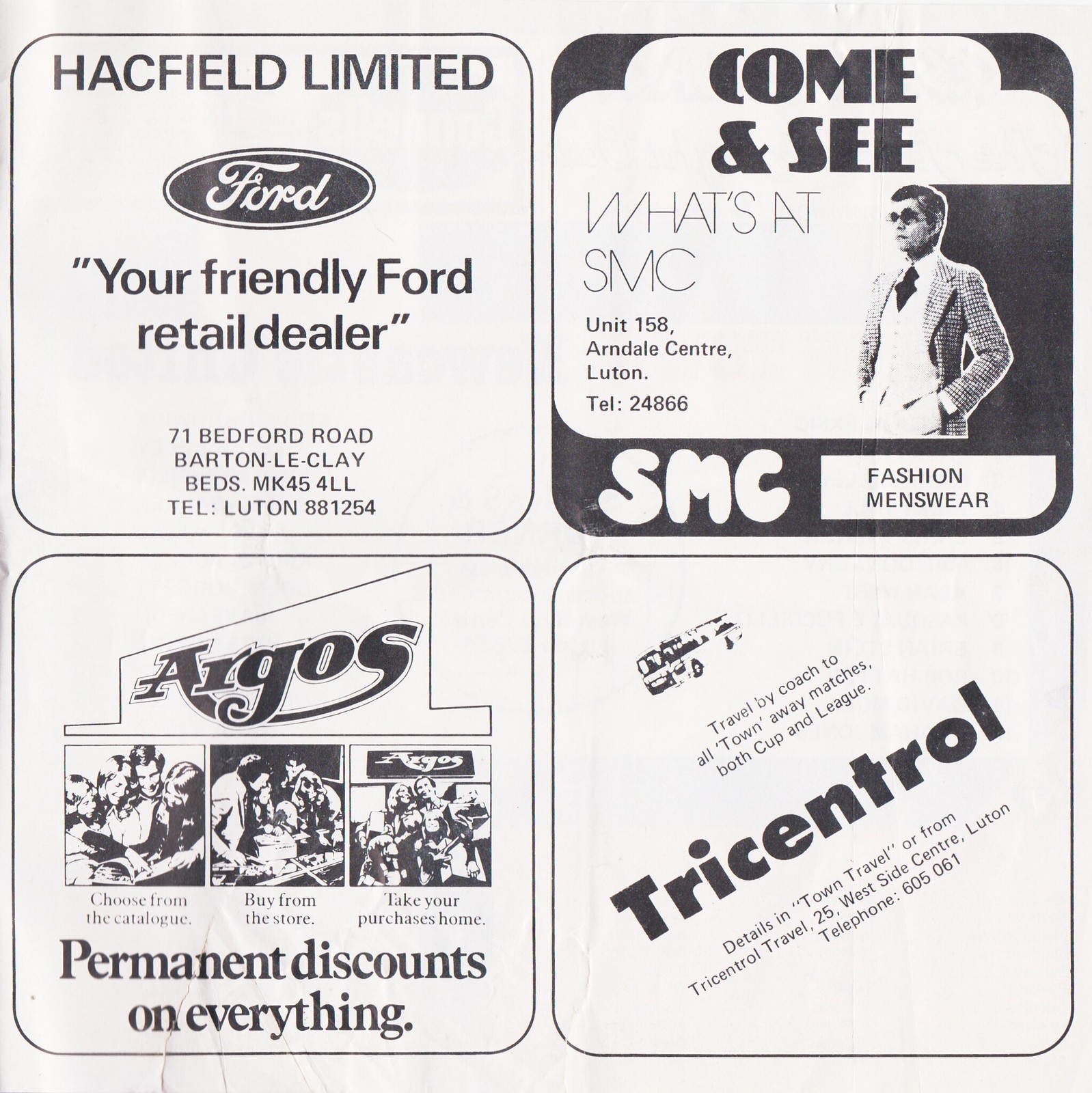This black and white image features four advertisements arranged in a grid with rounded corners, resembling a section of a vintage newspaper or magazine. Each ad occupies one square, with a clear emphasis on text and minimalistic black and white photos.

**Top Left:** The advertisement for Hackfield Limited prominently features the Ford Motor logo and reads, "Your friendly Ford retail dealer," offering services at 71 Bedford Road, Barton-le-Clay, Luton, England. Additional contact details are also included.

**Top Right:** An ad inviting customers to "come and see what's at SMC" showcases SMC Fashion Menswear at Unit 158, Arndale Center, in Luton. The ad includes a photo of a man in a suit, enhancing the menswear theme.

**Bottom Left:** The bottom left square displays an ad for Argos, highlighted by bold text at the top. It features a comic-strip-style illustration divided into three sections: "Choose from the catalog," "Buy from the store," and "Take your purchases home." The ad also mentions "permanent discounts on everything."

**Bottom Right:** The final advertisement promotes Tricentral with an image of a bus and text encouraging travel by coach to all town away matches, both cup and league. Details include the address at 25 Westside Center, Luton, and a telephone number for further inquiries.

This detailed arrangement of period advertisements captures the essence of mid-20th-century British retail and service promotion.